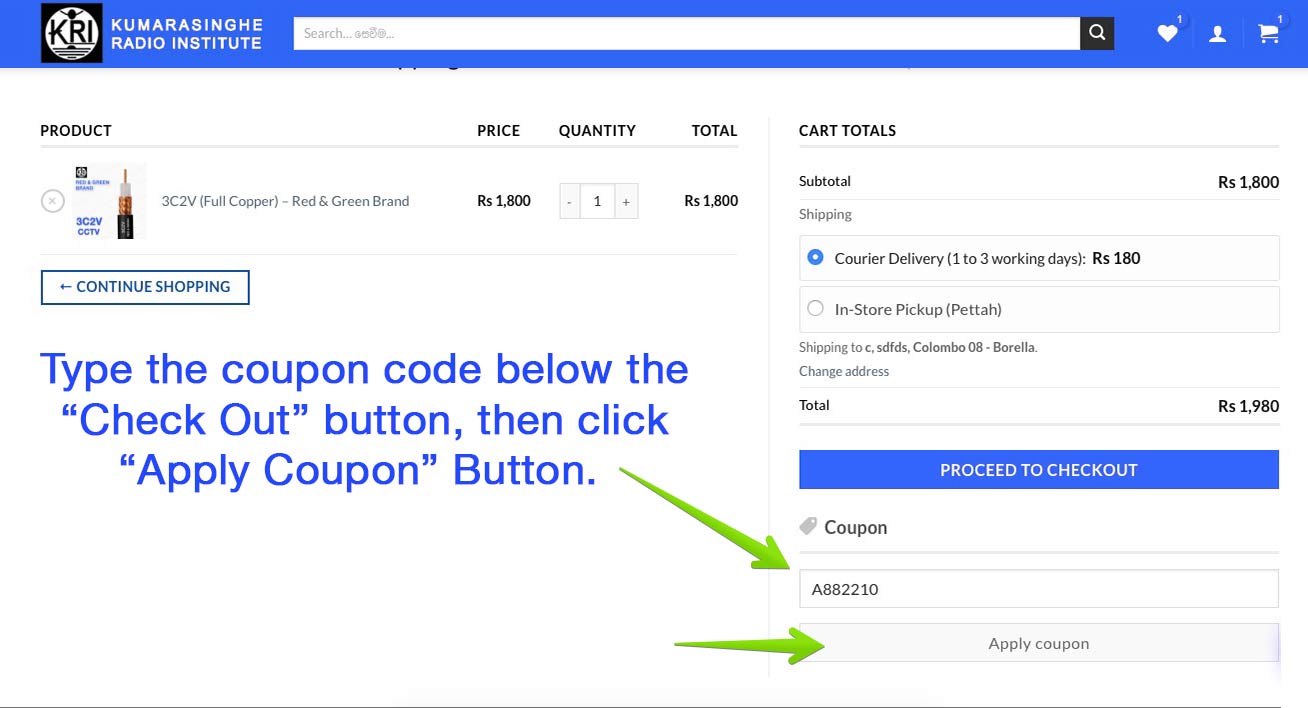This screenshot depicts a webpage from the Kumara Singh Radio Institute. In the upper left corner, there is a logo enclosed in a black square, featuring a round circle with the letters "KRI." To its immediate right, "Kumara Singh Radio Institute" is written in white text. A search bar follows, along with a black square icon displaying a white magnifying glass. Continuing to the right, there are three icons: a white heart next to the number 1, a profile icon, and a shopping cart icon with the number 1 indicating one item in the cart.

Directly below, a section labeled with "Product," "Price," "Quantity," "Total," and "Cart Totals" is arranged from left to right. An image displays the product: "3C2V full copper red and green brand," which appears to be a type of battery. The price is listed as RS-1800, with a quantity of 1, making the total RS-1800. Beneath this section, there is a "Continue Shopping" button in blue text.

Further down, prominently featured in large, bold blue text, are instructions for using a coupon code: "Type the coupon code below the checkout button. Then click apply button." Green arrows are used to point out both the space to enter the coupon code and the apply button.